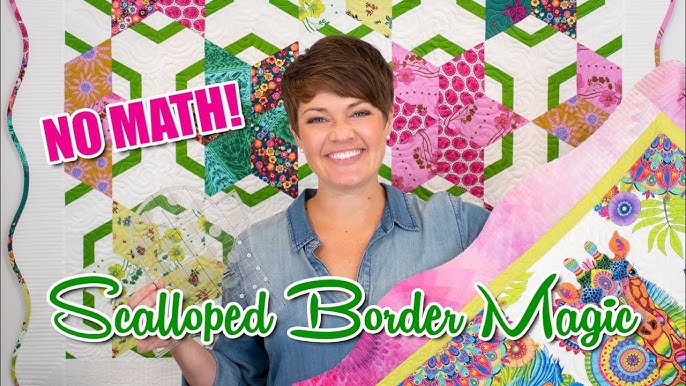The image appears to be a wide, horizontal screenshot of a webpage advertisement featuring a vibrant quilted background. The background showcases a white quilt adorned with a jagged, green horizontal line that undulates across its length. Interspersed across these lines are large, quilted stars in various colors, including pink, teal, and dark black with floral patterns. 

In the foreground, positioned slightly to the left, is an image of a woman up to her waist. She has light skin, short dark brown hair combed to one side, and is smiling at the camera. She appears to be in her 40s and is wearing a light blue, denim-like button-down shirt with the top buttons undone. She holds a clear object in her left hand, possibly a pattern or design sheet that blends into the quilted background.

Overlaying the image, in the top left corner, are the words "NO MATH!" in bold pink, all-capital letters. Below this, over the woman's chest in green text with a white outline, are the words "SCALLOPED BORDER MAGIC."